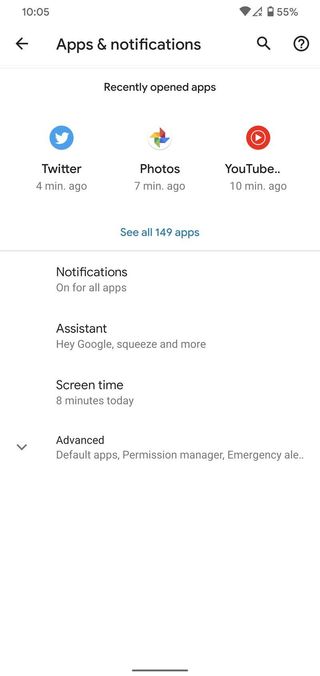This image captures the 'Apps & Notifications' settings screen on a smartphone. At the top, there is a back arrow indicating a way to return to the previous menu. Centrally located is the label "Apps & notifications." Directly beneath this, the section titled "Recently opened apps" lists applications used in the recent past. The first entry is Twitter, indicating it was opened 4 minutes ago, accompanied by the recognizable Twitter icon above the word "Twitter." Below Twitter, the Photos app shows it was last accessed 7 minutes ago, with its distinct icon placed above the text "Photos." The third app listed is YouTube, used 10 minutes ago, featuring the YouTube symbol above the text "YouTube." These three items are positioned side by side.

Below this section is an option labeled "See all 149 apps," allowing users to view a comprehensive list of installed applications. The next section states "Notifications on for all apps," signifying that notifications are enabled for every application. Further down, specific features and statuses include "Assistant," "Hey Google," and "Squeeze for more," suggesting voice assistant functionalities are mentioned. The "Screen time" indicates 8 minutes of usage for the day. The final option labeled "Advanced" suggests additional settings or information is available.